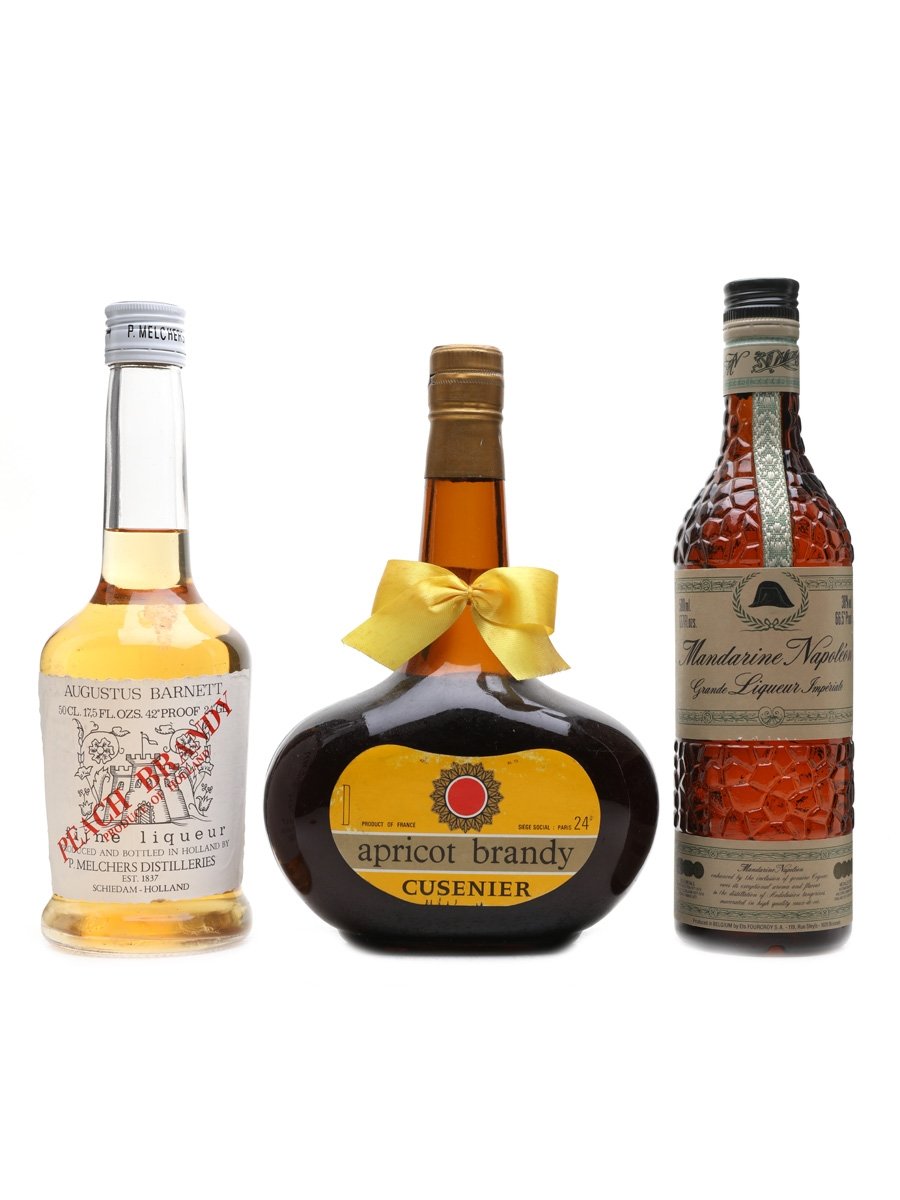This image features three distinct bottles of fruit-based alcoholic beverages set against a completely white background. Starting from the left, the first bottle is clear and contains a yellow liquid labeled "Peach Brandy" in diagonal red lettering, with a white cap. Moving to the center, the second bottle is darker and features an orange label with a gray stripe across the center, inscribed with "Apricot Brandy" and topped with a sun logo that has a red center. The neck of this bottle is adorned with a small yellow ribbon. Finally, the bottle on the right is a tall, thin, and textured clear bottle with a brownish-orange liquid inside, labeled "Mandarin Neptune Liqueur". Each bottle is distinctly styled but unified by their fruit-derived contents and elegant presentation.